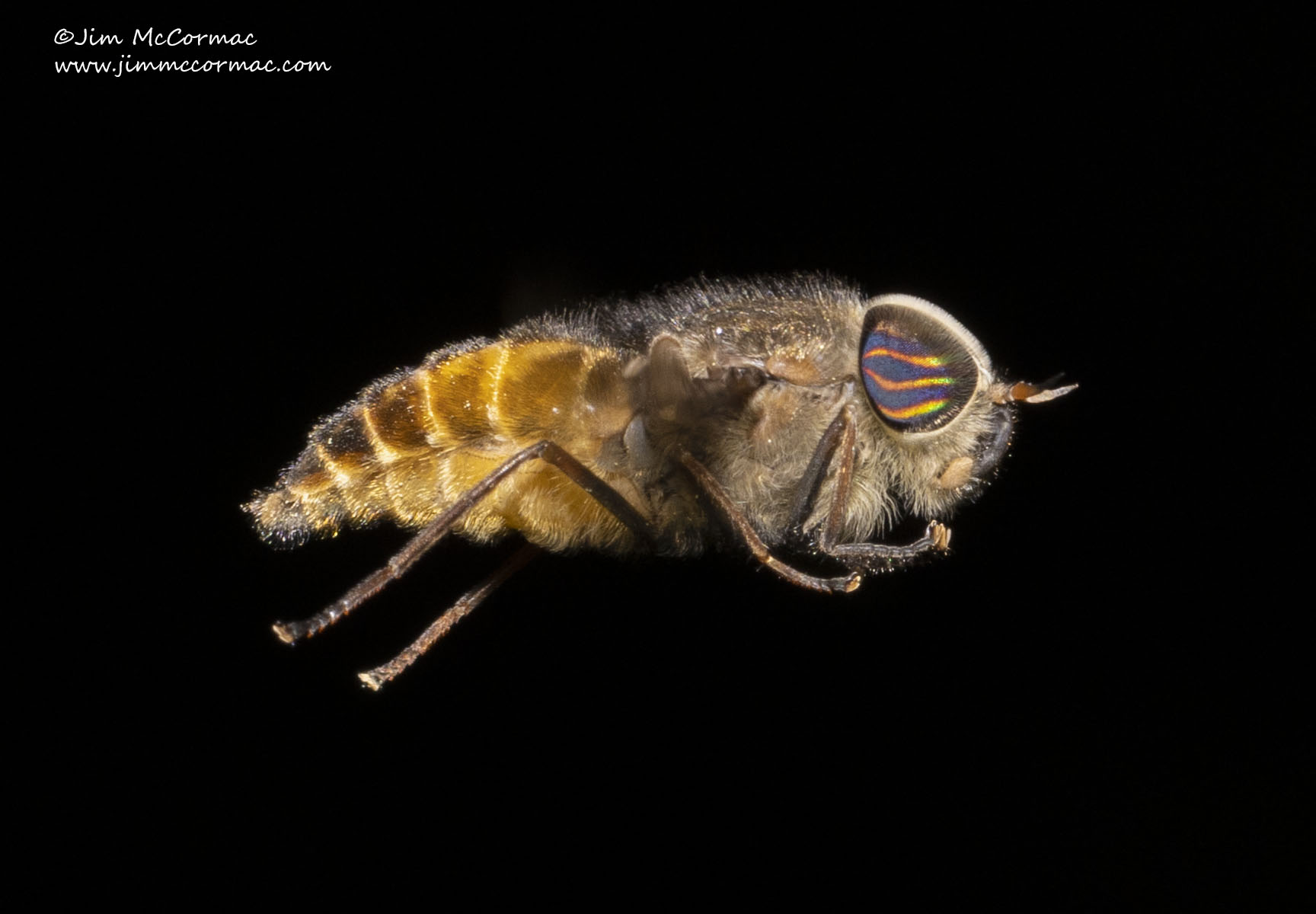The image showcases an extremely detailed, zoomed-in photograph of an insect that closely resembles a bee but lacks wings, suggesting it could be a wingless relative. The side view of the insect captures its head positioned toward the right with two distinctive horns protruding from its face. Set against a stark, black background, the insect's intricate features come to life. Its head, brown in hue, boasts large, bald eyes that are strikingly reflective with yellow streaks across a black outline. The body transitions from a brown thorax to a goldish-yellow tail, with numerous fine hairs visible across its form. Six legs are evident, further emphasizing the high level of detail captured in the photograph. The text "Jim McCormick" along with the photographer's website, "www.jimmccormick.com," is prominently displayed in the top left corner. The image's realism is heightened by the fur details and the mixture of colors, such as yellows and browns, that adorn the insect's body, making it so lifelike that it initially blurs the line between a photograph and a drawing.